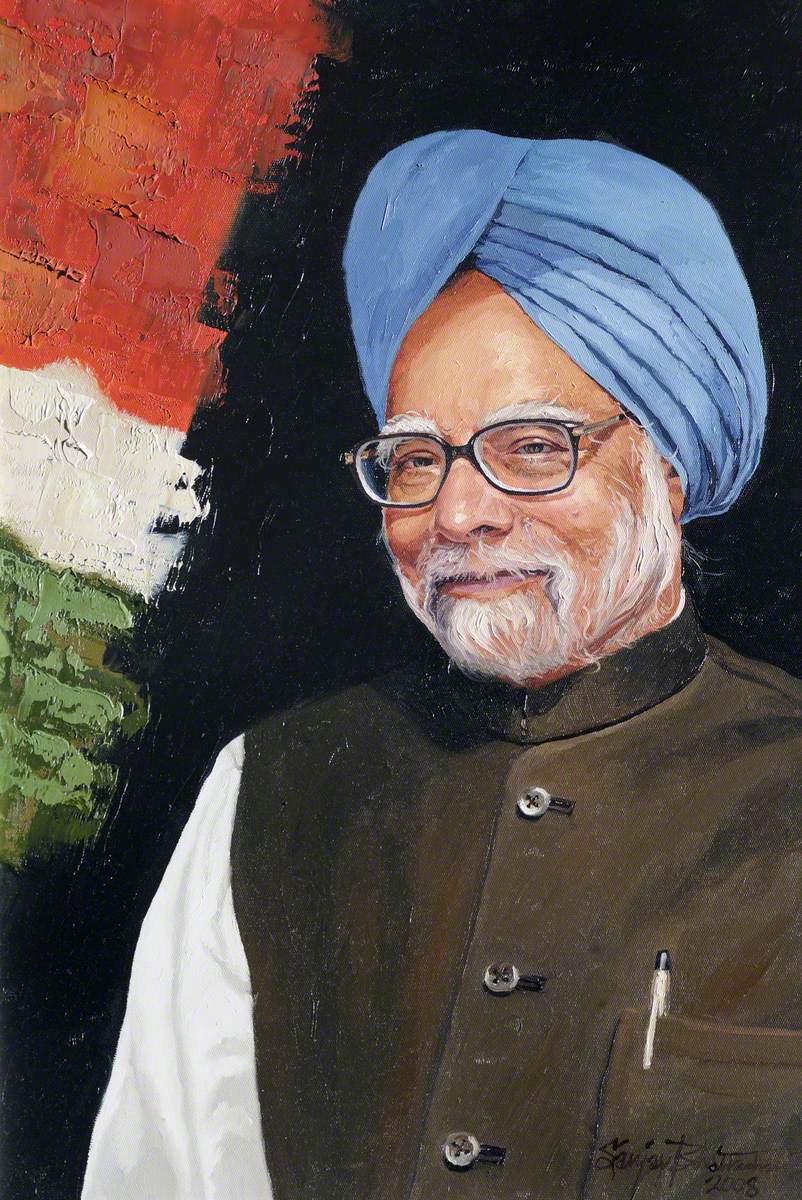The painting depicts an elderly man of Indian descent, distinguished by his medium blue turban, white eyebrows, goatee, mustache, and beard. He has a tan complexion, further emphasizing his advanced age. The man is wearing black, square-rimmed glasses and is smiling softly, with his eyes reflecting warmth and wisdom. His attire includes a white shirt beneath a dark brown, button-up vest that features a high collar covering much of his neck. A pen is neatly tucked into the vest pocket to his left, corresponding to the right side of the image. The background primarily displays a painted black brick wall with red, white, and green sections, evoking a crayon-like, possibly flag-inspired, design. The overall composition highlights the man’s serene and pleasant demeanor as he gazes into the distance.